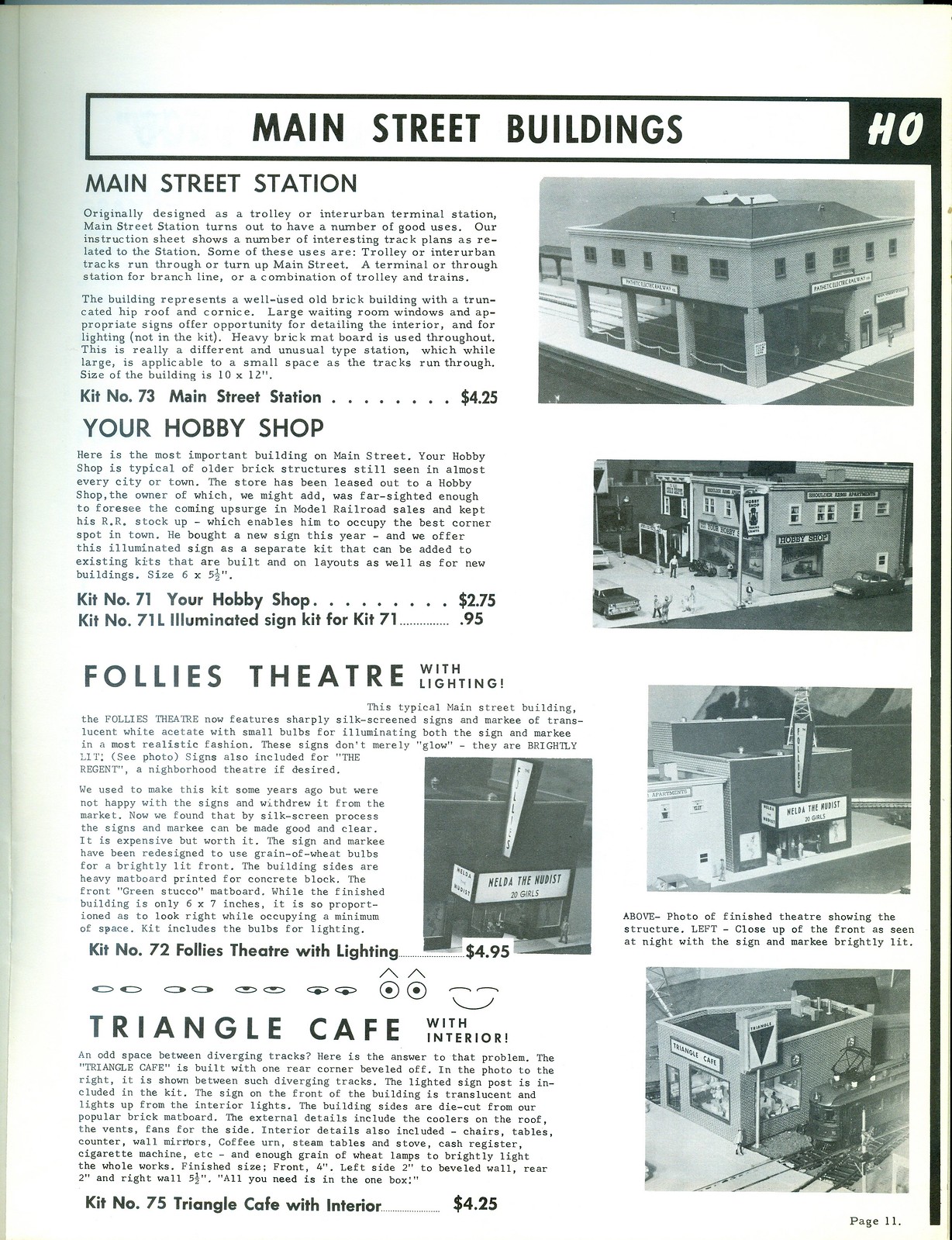The image is a black and white magazine page, likely page 2 of the publication, designed for a vintage print aesthetic. The page is outlined with a black rule and features the heading "MAIN STREET BUILDINGS" in bold, black capital letters within a white banner bordered in black. In the top right corner of this header, there is a black rectangle with "HO" in white bold italic letters, indicating the scale for model train settings.

Below the header are four sections, each dedicated to a different building with associated photographs and descriptive text:

1. **Main Street Station**: A descriptive paragraph sits beneath the title, though it's too small to read clearly. A black and white photograph of the station from a front-right corner perspective is provided beside this text. Below the paragraph, it states "KIT NO.73 Main Street Station... $4.25."

2. **Your Hobby Shop**: Following the same format, a detailed paragraph about this building is present but almost illegible due to small font size. There is a black and white photograph on the right showing a similar perspective of the shop. Pricing details at the bottom read "KIT NO.71 Your Hobby Shop... $2.75" and "KIT NO.71L Illuminated sign for KIT 71... $0.95."

3. **Folly Theater with Lighting**: This section includes a detailed write-up and multiple black and white photographs of the theater beside the text. Pricing at the bottom states "KIT NO.72 Folly Theater with Lighting... $4.95."

4. **Triangle Cafe with Interior!**: The text describing this building is followed by a photograph, again in black and white. At the bottom, it notes "KIT NO.75 Triangle Cafe with Interior!... $4.25."

All photographs and descriptions are presented in a portrait-oriented layout, with the descriptive text on the left and images on the right. The overall style echoes vintage photography and print publication, aimed at enthusiasts of HO scale model train setups.